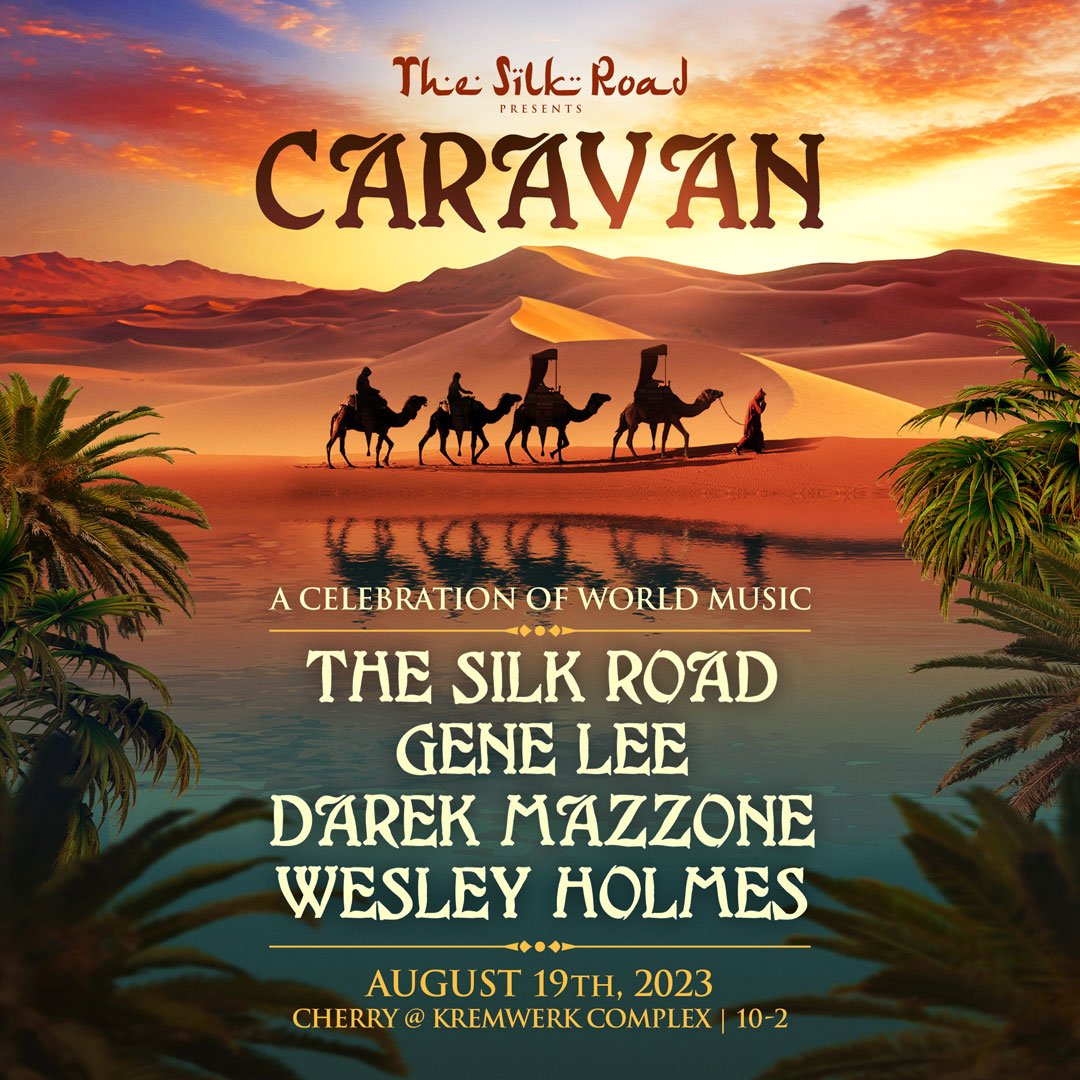The poster promotes a music festival titled "The Silk Road Presents Caravan: A Celebration of World Music." It depicts a desert scene with vibrant orange and yellow skies, accented by dark red clouds hovering over expansive sand dunes. In the foreground, silhouettes of five camels, each ridden by a man, traverse the desert. One of the men stands ahead, leading the procession by holding a rope tied to the lead camel. Notably, the first two camels have coverings to shield their riders from the sun's harsh rays. Below this evocative image, information about the event is displayed: 

- "The Silk Road Presents Caravan" is written in prominent brown text.
- "A Celebration of World Music" is rendered in white, with a gold line underneath.
- Following this, the names "The Silk Road, Gene Lee, Derek Mazzone, Wesley Holmes," also in white, are listed above another gold line.
- The date "August 19th, 2023" is highlighted in gold, accompanied by details stating "Cherry at Kremwerk Complex, 10-2."

The striking visuals and detailed text together effectively convey the essence and grandeur of this international music celebration.